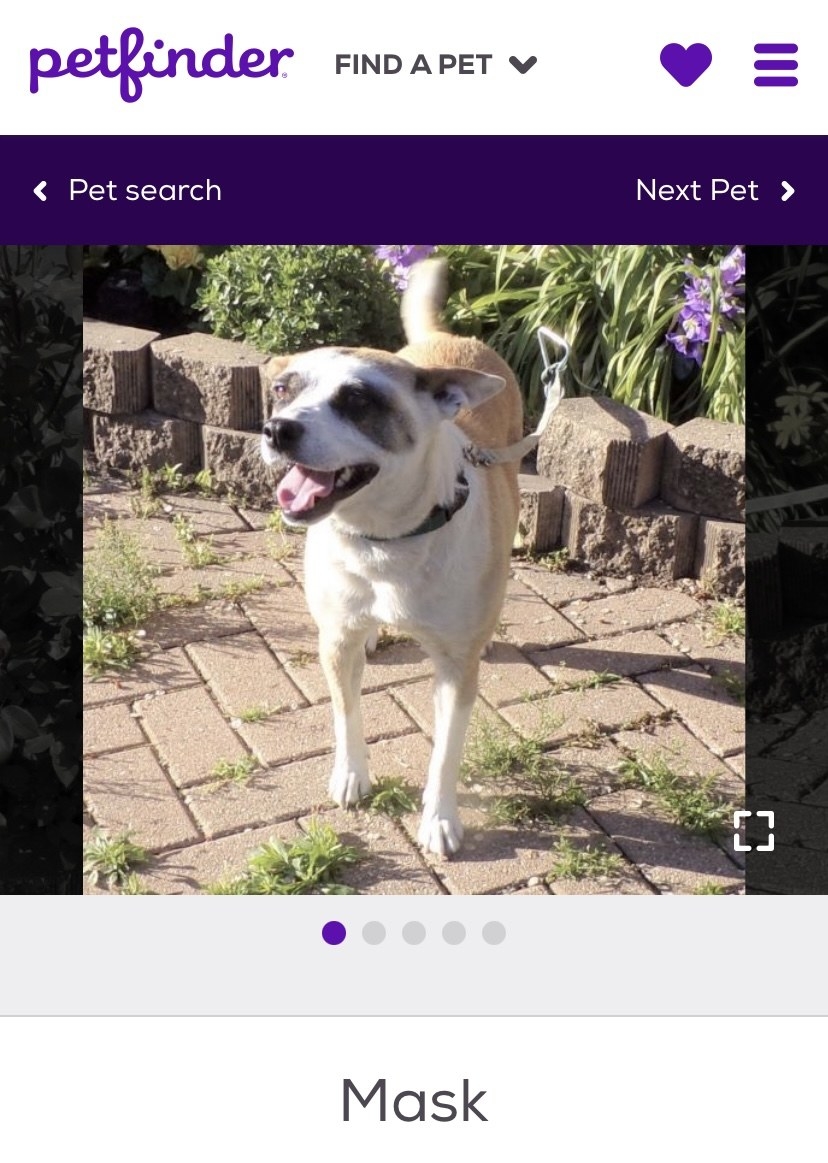This is a screen capture from the Petfinder website, prominently featuring the Petfinder logo in the upper left corner, crafted in a purple script font. To the right of the logo, the words "Find a Pet" are displayed alongside a down arrow.

At the image's center is a photograph of a dog, captured from a three-quarter view as it looks to the left. The young dog has an open mouth, suggesting a happy demeanor. Its coat is primarily white on the chest, with brown fur covering its back and a distinctive black patch around its left eye, which hints at its playful name, "Mask." Although the right eye is less visible due to the sunlight casting shadows from the left, the light hints at a similar black marking on that eye as well.

The dog, appearing healthy and vibrant, is estimated to be around two to three years old. It is wearing a leash that connects to a post situated in a garden, visible in the background.

Text elements are strategically placed throughout the upper portion of the screen capture. "Pet Search" is accompanied by a left-pointing arrow, while "Next Pet" appears with a right-pointing arrow. At the bottom of the image, a series of five dots serves as navigation indicators, with the leftmost dot highlighted in purple, signifying the current image in a scrollable series. To the right of the dots, the remaining four are gray, indicating additional images available for viewing.

Lastly, the name "Mask" is displayed below the image, likely indicating the dog's name, which fits with its distinctive facial markings resembling a mask. 

This detailed screen capture from Petfinder highlights "Mask," a charming young dog ready for adoption.